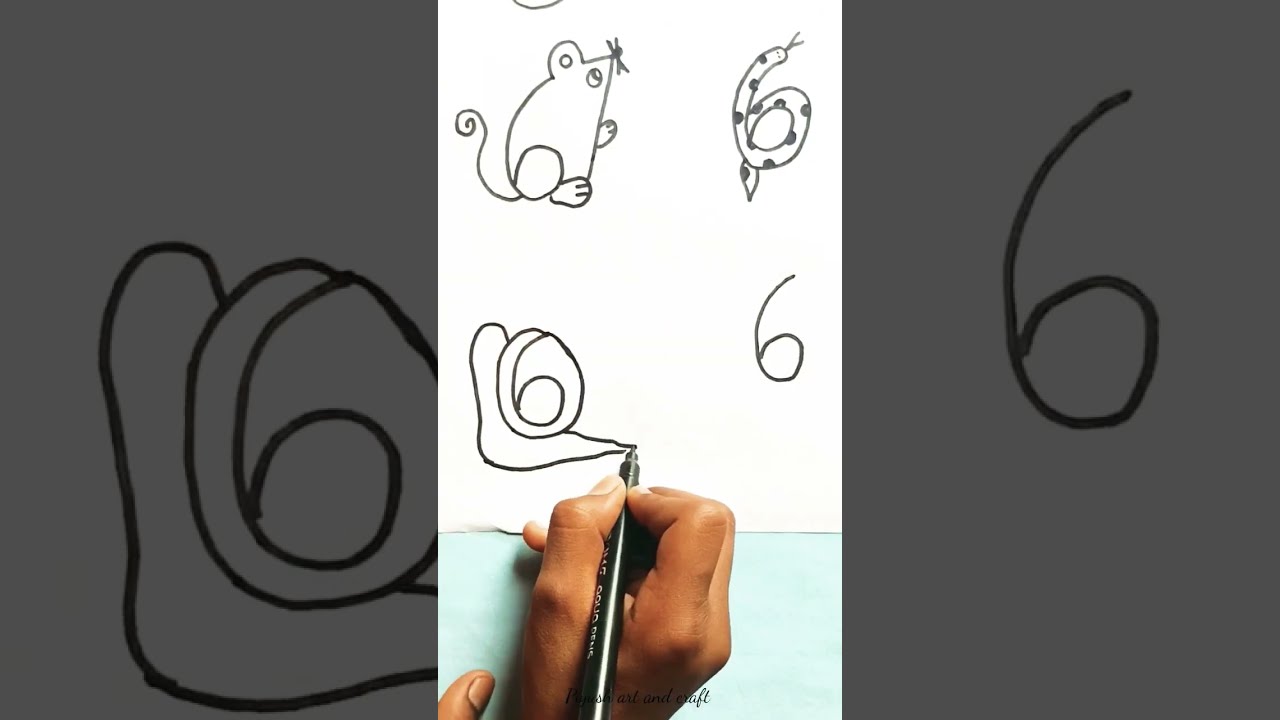The image captures a person with a darker skin tone using their right hand to draw detailed illustrations with a black plastic pen on white paper. The drawing process revolves around creatively transforming the number six into various objects. In the top left, the number six has been ingeniously turned into a mouse, with the round part of the six forming the mouse’s rear end and added features like a curly tail, feet, an eye, a nose, and an ear. To the right of this is another transformation, where the six becomes a snake with an extended tail. Below the mouse, the number six is being shaped into a snail, utilizing the loop of the six as the snail's shell and drawing the body around it. There's also an untouched number six depicted beside these illustrations, ready for transformation. The entire drawing is set against a plain white background, with the bottom part of the image showcasing a light blue hue as part of the drawing workspace.